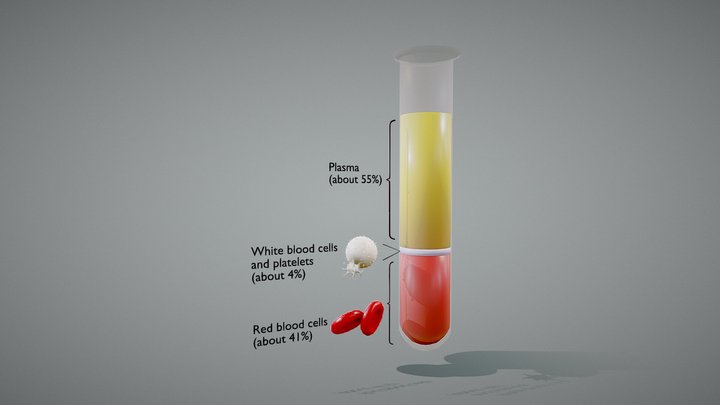This is a diagrammatic image of a laboratory test tube segmented into three distinct layers of blood components, set against a gray background. The top two-thirds of the test tube contains a yellow liquid labeled "plasma," approximately 55% of the total volume. Below the plasma, there is a narrow white band representing "white blood cells and platelets," making up about 4% of the content. The bottom section, comprising about 41% of the tube, is filled with a red liquid labeled "red blood cells." Each section is annotated with lines pointing to descriptive text, including informative labels and small images of the represented blood cells: a white ball for white blood cells and two red blood cells for the red layer. The test tube appears more like an illustrative diagram rather than a photorealistic image.